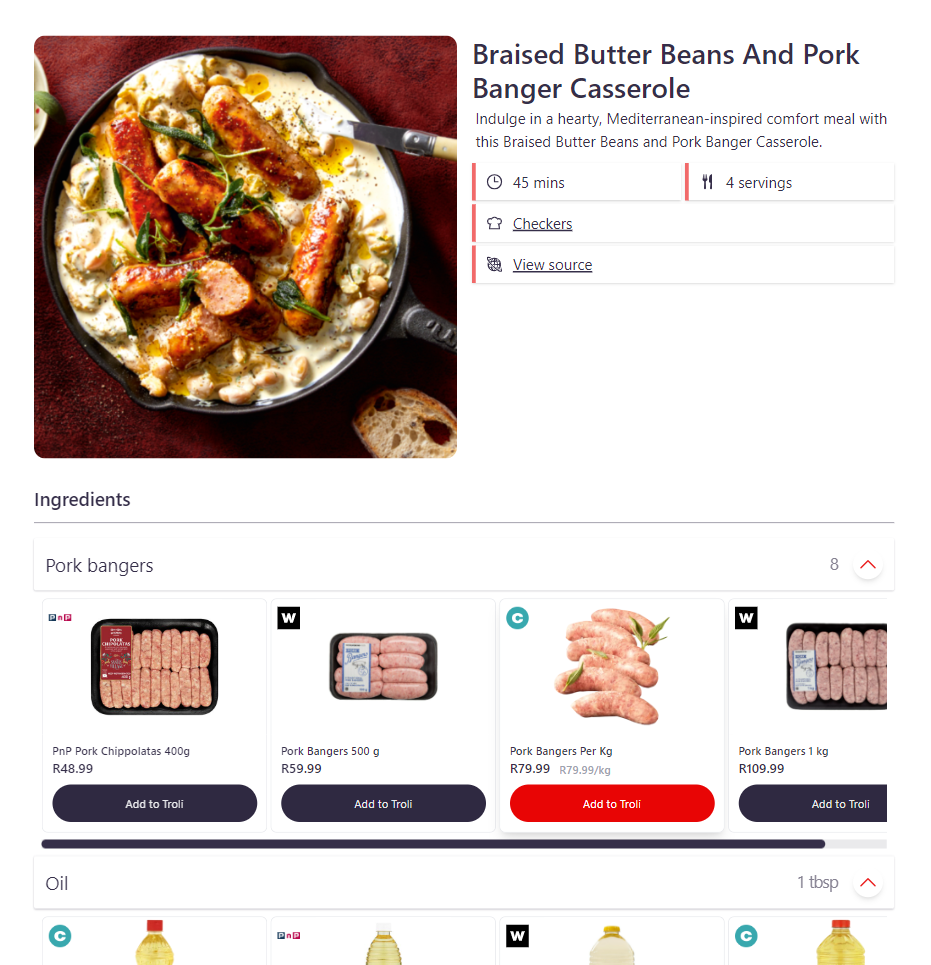The image appears to be a screenshot from a recipe app or website featuring a detailed recipe for a Mediterranean-inspired dish. At the top left, there's a large photo showcasing a pan full of sausages, possibly immersed in a bean concoction. To the right of the image, a text description reads: "Braised Butter Beans and Pork Banger Casserole." Following the image, a brief description entices the viewer: "Indulge in a hearty Mediterranean inspired comfort meal with this braised butter beans and pork banger casserole."

Beneath the description, a table provides vital information about the recipe: the estimated cooking time of 45 minutes, and the serving size of four portions. 

Spanning the width of the screen below the introductory section, there’s a bold heading that says "Ingredients," underlined by a gray bar. The listed ingredients start with "Pork bangers" followed by an '8' aligned to the right, accompanied by a small upward arrow within a circle. 

Further down, several product images related to the recipe are displayed: "PnP Pork Chipolatas 400 grams," "Pork bangers" with an image above it, and "Pork Bangers per kg." The detailed layout and the vivid pictures make it easy for users to visualize and gather the necessary ingredients.